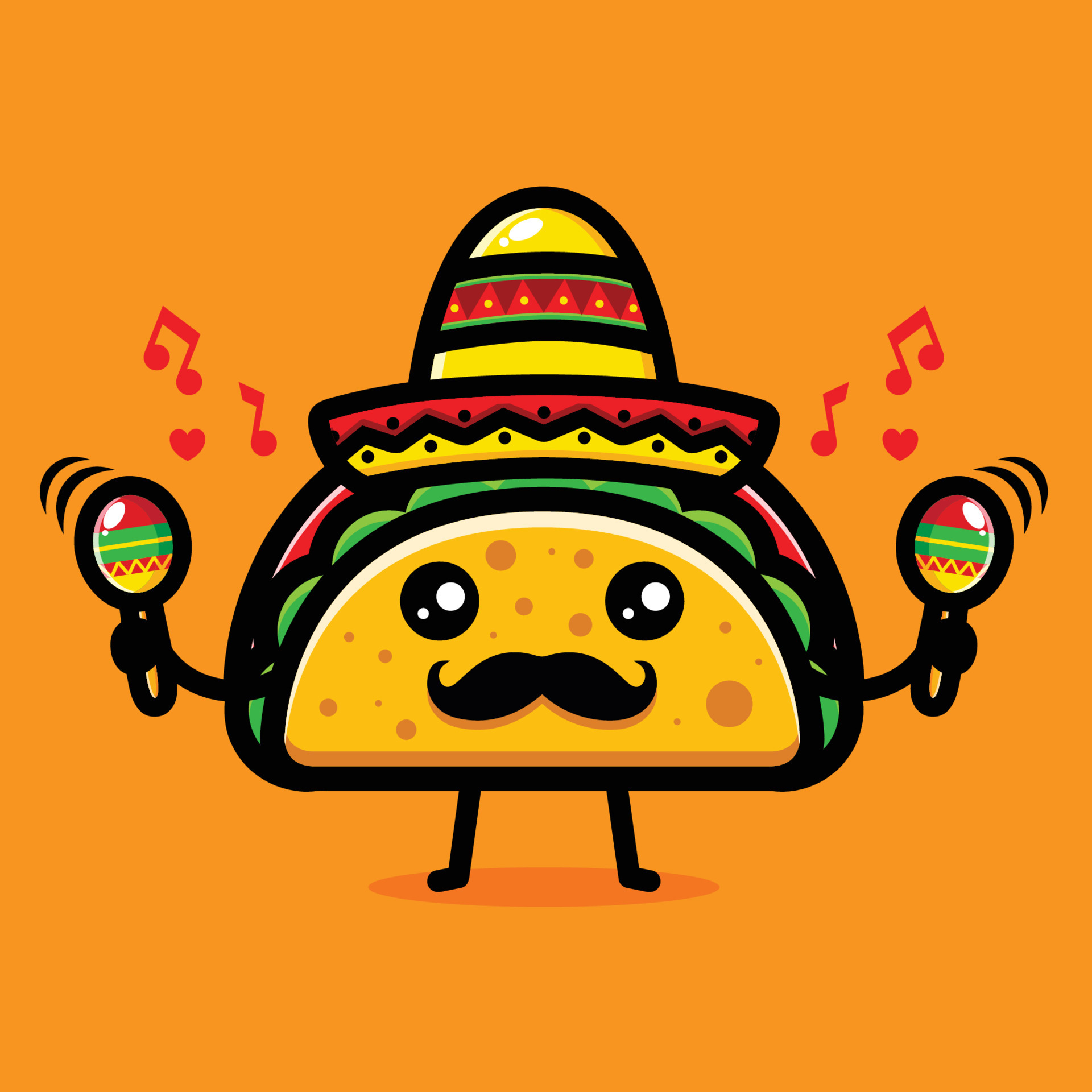The image is a clipart of a taco standing on a dark orange oval against a dark orange background. The taco has a face with black eyes and a black mustache, and it features stick-figure-like black legs and arms. The arms are holding maracas in red, green, and yellow, with red musical notes and hearts emanating from them, along with action lines indicating the maracas are being shaken. The taco is adorned with a sombrero, which is yellow with a red and green triangle stripe pattern. The taco filling includes light orange for the tortilla, green lettuce, and red elements that could be either tomato or meat.